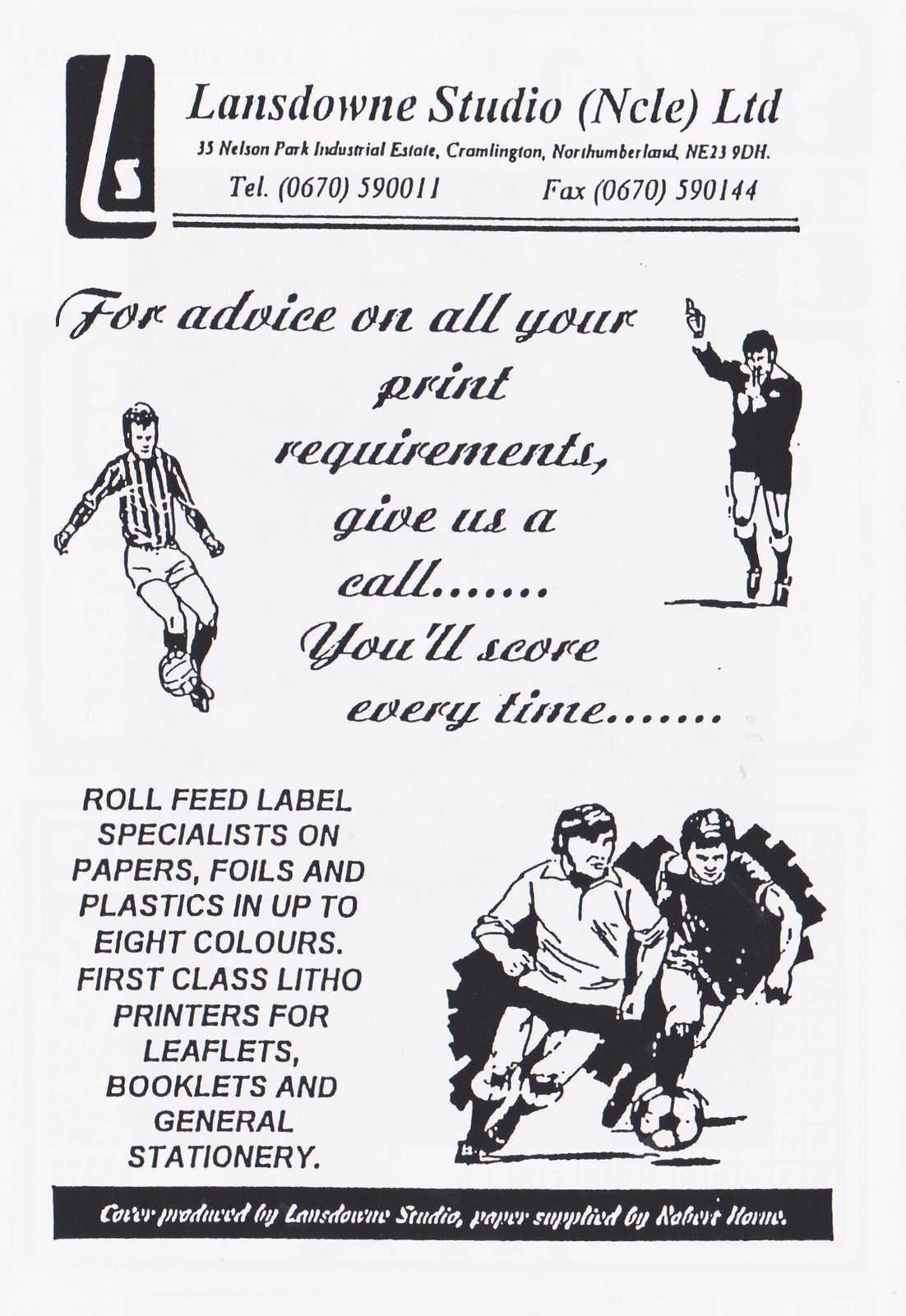The image is an old black-and-white advertisement, possibly torn from a pamphlet or newspaper, for Lansdowne Studio, LTD, located at 35 Nelson Park Industrial Estate, Cramlington, Northumberland. The ad features multiple hand-drawn illustrations of people playing soccer, including a referee kicking a ball, players running towards it, and an official blowing a whistle. The advertisement promotes the company's services with text stating, "For advice on all your print requirements, give us a call. You'll score every time." It lists a telephone number (0670-590011) and a fax number (0670-590144). The ad highlights Lansdowne Studio as specialists in roll feed labels on papers, foils, and plastics in up to eight colors, and notes their expertise in first-class lithographic printing for leaflets, booklets, and general stationery. A banner at the bottom mentions, "Cover produced by Lansdowne Studio, paper supplied by [unreadable text]."